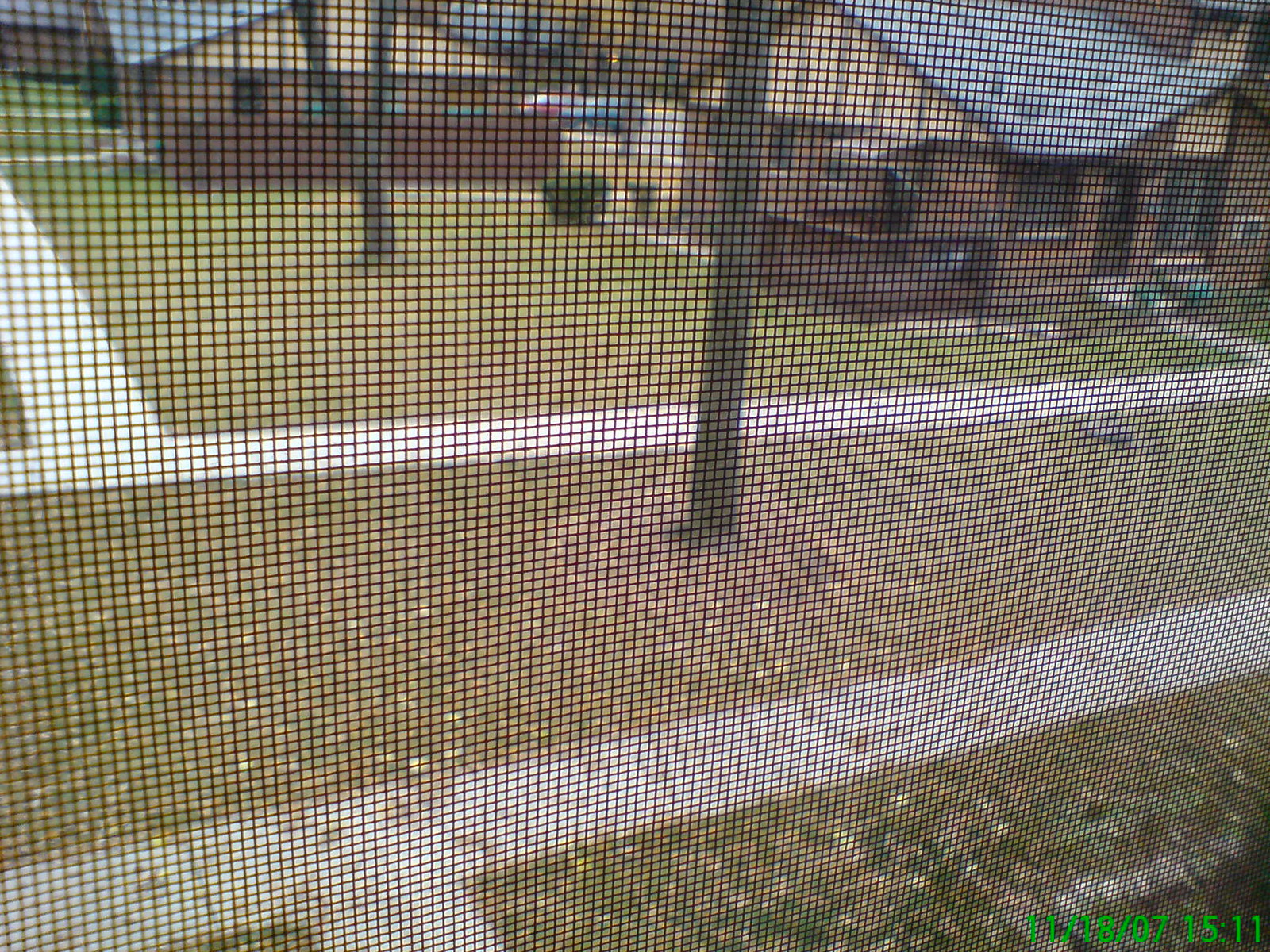The image depicts a scene captured through a screen window, evident by the black grid overlay throughout the photograph, giving the impression of a security camera feed. The timestamp in the bottom right corner reads "11/18/07 15:11" in green digits, indicating the photograph was taken on November 18, 2007, at 3:11 PM.

The setting is a quaint neighborhood sidewalk in view of the camera, revealing multiple parallel sidewalks separated by strips of grass. The closest sidewalk runs alongside a curb and the street, flanked by a verdant patch of grass with trees whose trunks are surrounded by dirt and scattered, light brown autumn leaves.

In the upper part of the image, two one-story brown houses with light gray roofs can be seen. Each house features a small brown deck and windows with dark brown frames. Leading up to these houses are light cream-colored pathways. The overall scene is a tranquil residential area, captured on a serene fall day.